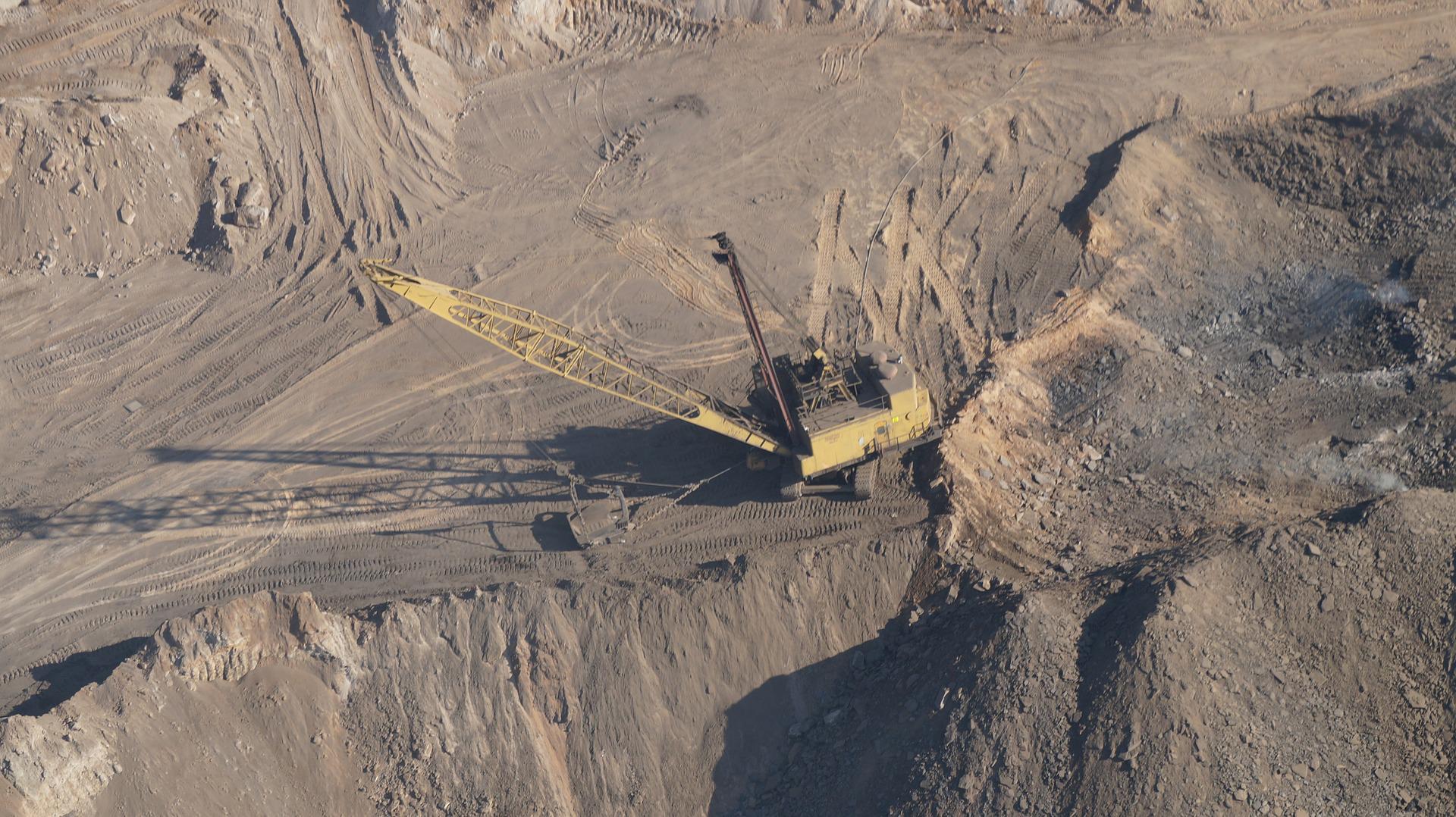This detailed aerial image captures a vast mining or excavation site, dominated by a landscape of dark dirt, rock, and rugged cliffs. Central to the scene is a prominent yellow excavator, equipped with an extended crane-like arm, which features a large jaw mechanism designed to dig and lift soil or ore from the ground. The excavator casts a distinct shadow on the ground, indicating a bright, sunny day. Surrounding the excavator, the terrain shows signs of substantial clearing, particularly evident on the right-hand side where the ground appears smoother and lighter.

In the foreground, there appears to be a deep pit, where the excavator operates, suggesting ongoing excavation activities. This pit contrasts with the flat, undisturbed terrain on the right edge of the image, which is marked by darker rock. Cutting across the middle of the scene is a well-traveled road, likely used for transporting materials away from the site, possibly by dump trucks. This road is a key feature, providing a clear division between the cleared pit area and the rest of the landscape. Additionally, in the top-left corner of the image, a lighter road extends off the frame, showing tire tracks that suggest regular use. 

In the background, the excavated land shows alternating bands of cleared and untouched areas, along with accumulated dirt mounds. The overall composition of the image highlights both the scale and activity of the mining operation, with the central yellow excavator serving as a focal point amid the expansive excavation site.